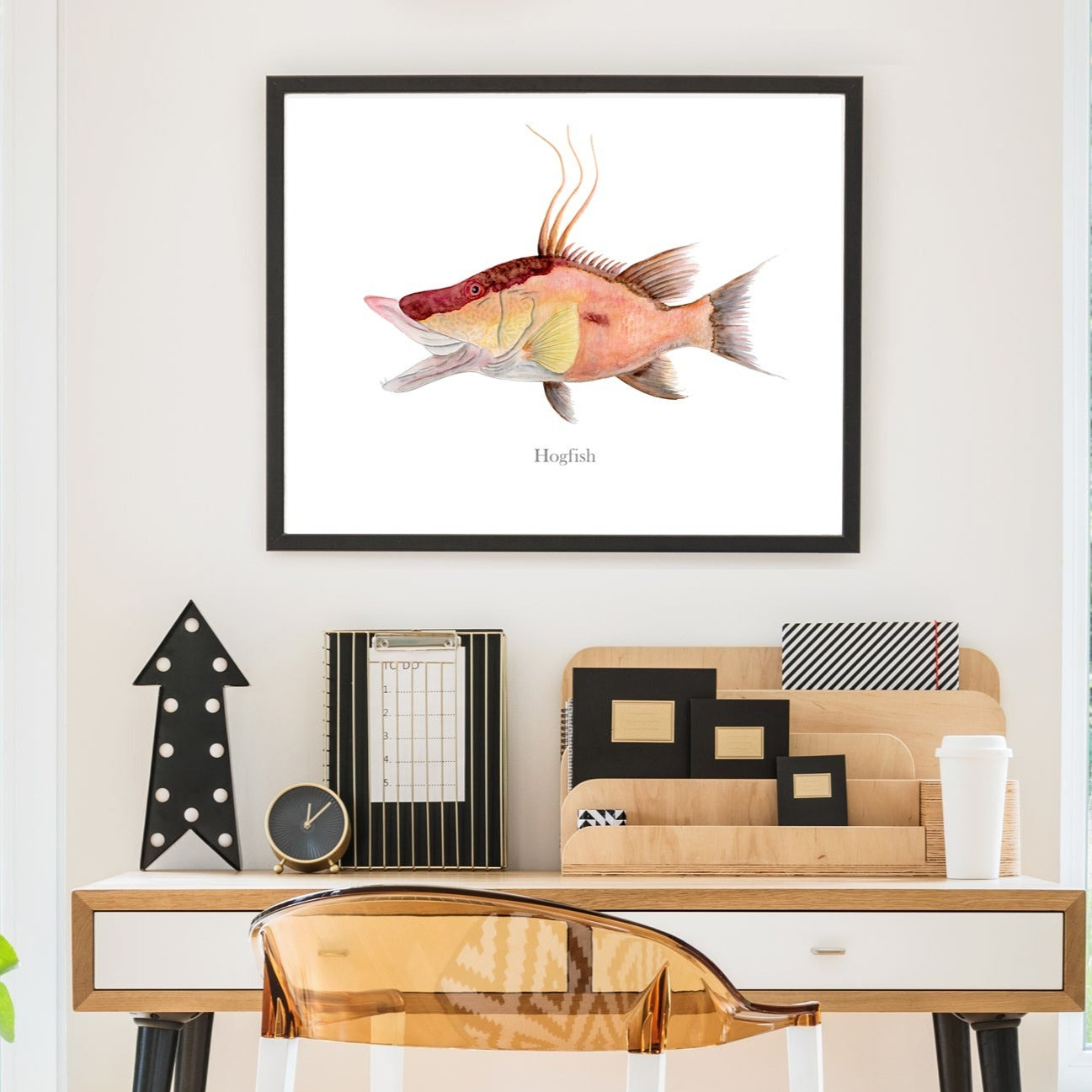This brightly lit photograph captures a close-up view of a stylish office desk setup. At the center of the image is a tan wooden desk with four black legs and two long rectangular white drawers featuring elegant gold handles. Positioned in front of the desk is a modern, transparent amber acrylic chair with white legs, adding a contemporary touch to the space.

On the desk, an arrangement of various items brings a sense of organization and purpose. To the right, a black and gold clock without numbers stands next to an organizer filled with papers and stationery. A white disposable coffee cup with a lid sits nearby. On the left side of the desk, a blue clipboard with white vertical lines is neatly placed beside a black arrow adorned with white lights pointing upward, creating a focal point against the wall.

Above the desk, a wall-mounted picture of a hogfish draws attention with its detailed, colorful illustration. The fish, depicted in shades of pinky-red, red, and orange with yellow fins and three long tendrils, is framed by a black border against a clean white background. The word "hogfish" is inscribed beneath the vivid image, completing the well-composed and thoughtfully designed workspace.